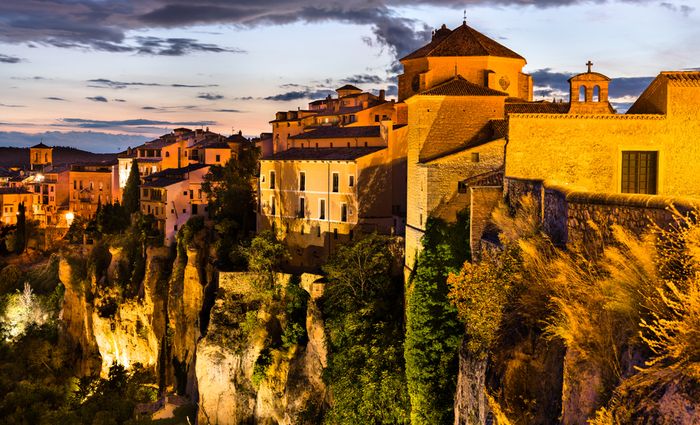This image presents a breathtaking, almost surreal scene of a cliffside village at twilight, possibly either dawn or dusk. The sky is a palette of light dusky blue with dark gray clouds, accented by a thin ribbon of pink along the horizon. The village clings precariously to the edge of a golden-hued cliff, which is dotted with a variety of green foliage and patches of golden grass. The buildings, evocative of Mediterranean architecture, are bathed in a yellow-golden light, perhaps due to the reflection of the sunrise or sunset. They are crafted from stone or stucco, with brown roofs, and one structure prominently features a cross, indicating a church. No people or text are visible, emphasizing the serene and somewhat mysterious atmosphere. The overall composition skillfully highlights the interplay of natural beauty and human ingenuity in harmony with the rugged landscape.